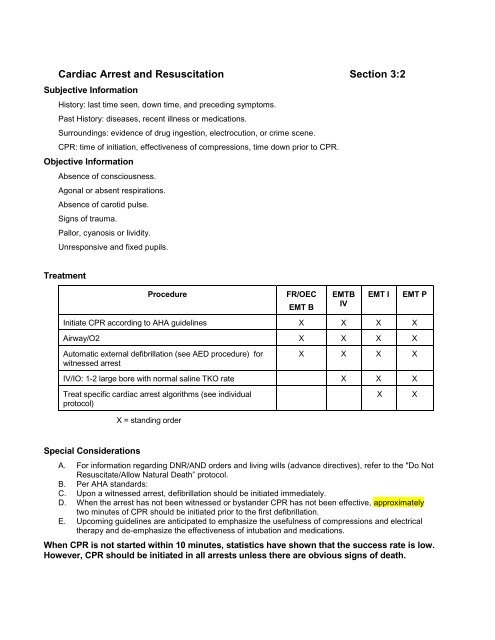This is an information sheet titled "Cardiac Arrest and Resuscitation, Section 3.2." It features a crisp white page with black print. The document is divided into four distinct sections: Subjective Information, Objective Information, Treatment, and Special Considerations. Each section provides detailed guidance pertinent to its heading. Notably, the word "approximately" is highlighted in yellow under Special Considerations bullet point D. The Treatment section includes a detailed chart with five rows and four columns, offering procedural instructions and designated spaces or marks for each procedure. The print throughout the page is quite fine, with detailed but small text under each heading.